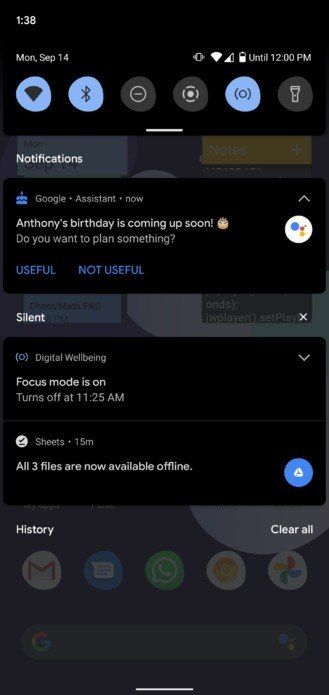This image, captured on an iPhone, showcases a detailed screen interface. On the upper right side, the time is displayed as "Until 12 p.m." The battery icon indicates it is about 75% charged, and the connection strength is very strong. The date is prominently shown as Monday, September 14th. At the top of the screen, there are six icons: three blue and three black. Below these icons is a white line, dividing the top section from the rest of the content.

To the left of the screen, a gray box labeled "Notifications" is prominently visible. To the right, there is another label "Notes," but it is grayed out, indicating it is not currently active. Underneath these labels, there is a prompt from Google Assistant stating, “Anthony's birthday is coming up soon,” accompanied by an icon and a large, colorful circle. It asks, "Do you want to plan something?" with options "Useful" and "Not useful" presented in blue beneath the query.

Further down the screen, there is a thin box labeled "Silent." Below it, the screen indicates that "Digital Well-being focus mode is on" and will turn off at 11:25 a.m. Another notification reads, "Sheets - 15 minutes: All three files are now available offline," marked with a blue circle next to this information.

At the bottom of the screen, there is a section labeled "History," accompanied by five small icons. The screen offers two options: "History" on the left side and "Clear all" on the right side.